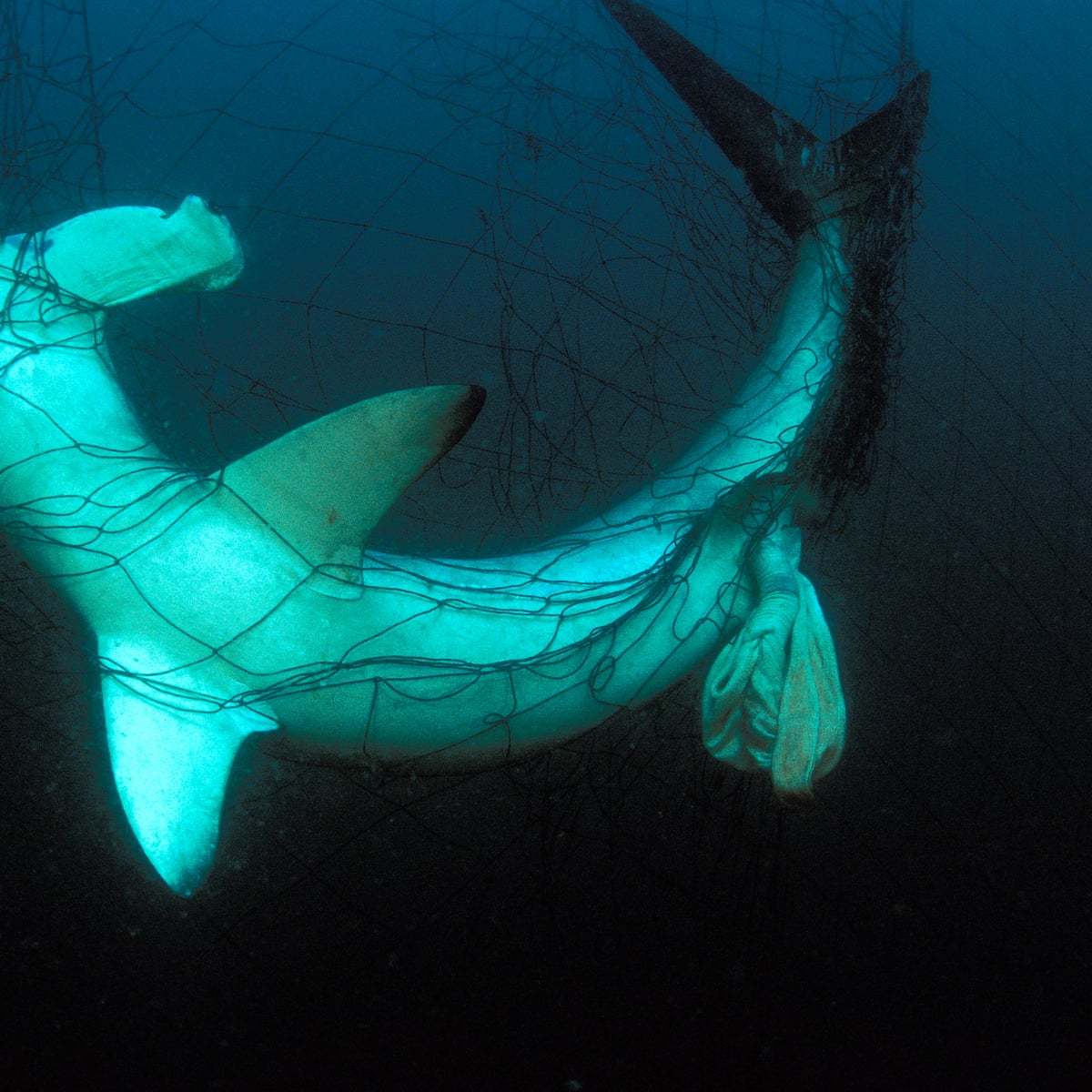The image captures a poignant underwater scene featuring a shiny, pale green hammerhead shark ensnared in a black fishing net. The shark, noticeable for its uniquely shaped head with rectangular extensions housing its eyes, is struggling futilely within the net. The netting is tightly wound around its body and tail, with strands even encircling its neck, accentuating the tragic entrapment. The dark black bottom of the scene contrasts sharply with the medium-tone blue upper background, emphasizing the shark’s predicament in the depths of the ocean. The visible fins on either side, the dorsal fin, and the curved body of the distressed shark highlight its large size and strength, now subdued and immobilized by the net, conveying a sense of sadness and desperation.